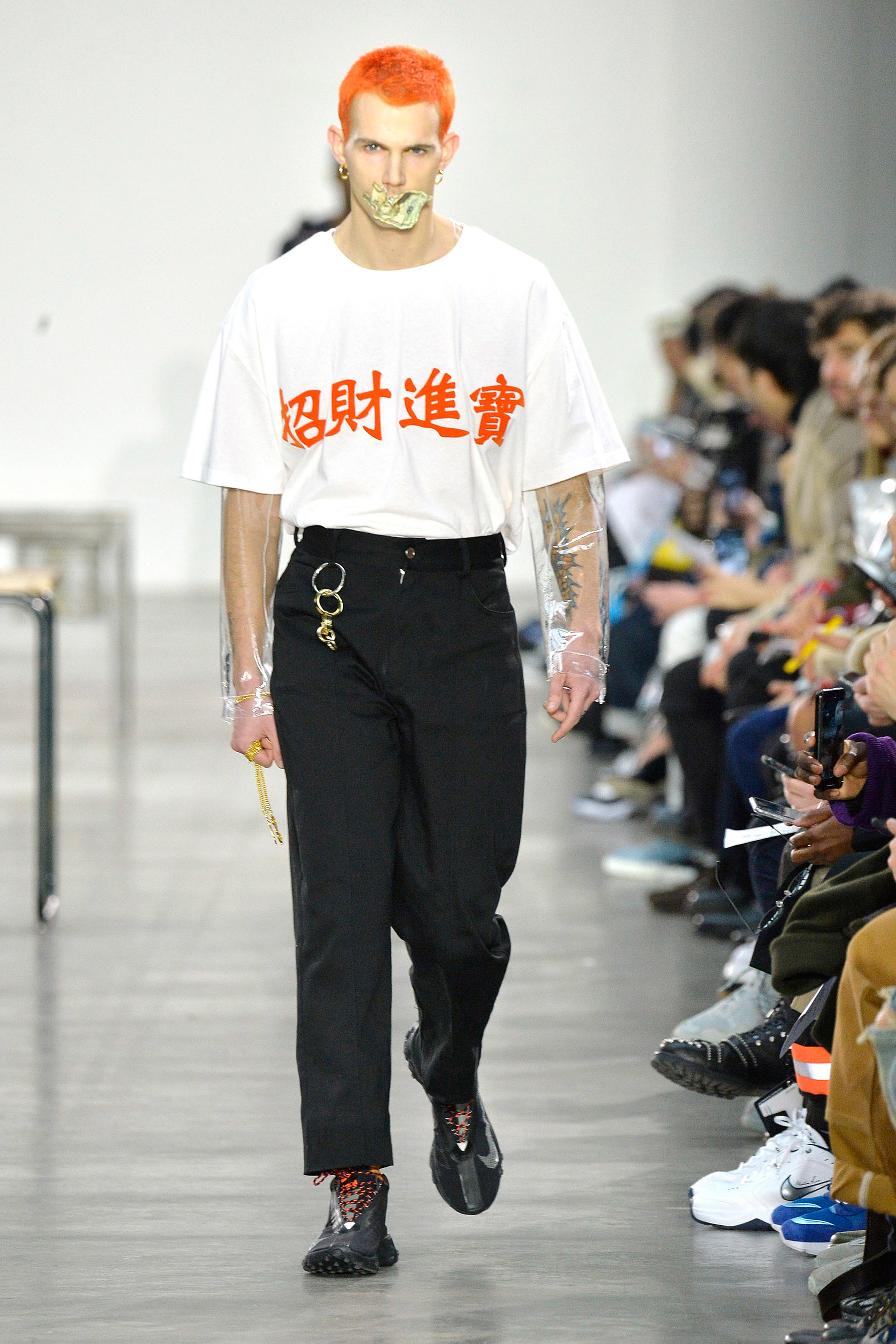A young Caucasian male model with bright orange hair and gold circular earrings is making a stride down an eccentric, concrete runway, typical of a fashion show. His mouth is conspicuously covered with what seems to be cash, perhaps taped or stuck to prevent him from speaking. He dons a white short-sleeve shirt featuring four bold orange Chinese characters, matching his hair color. Intriguingly, clear plastic sleeves extend from beneath or are attached to this white shirt, covering his arms down to his hands. He pairs this with black pants, adorned with a gold chain that he holds in one hand and multiple rings or key holders hanging from the belt loops. His black athletic shoes, sporting orange shoelaces, complete the striking outfit. The runway is flanked by an audience busily taking photos and notes, clad in fashionable outfits and sneakers.